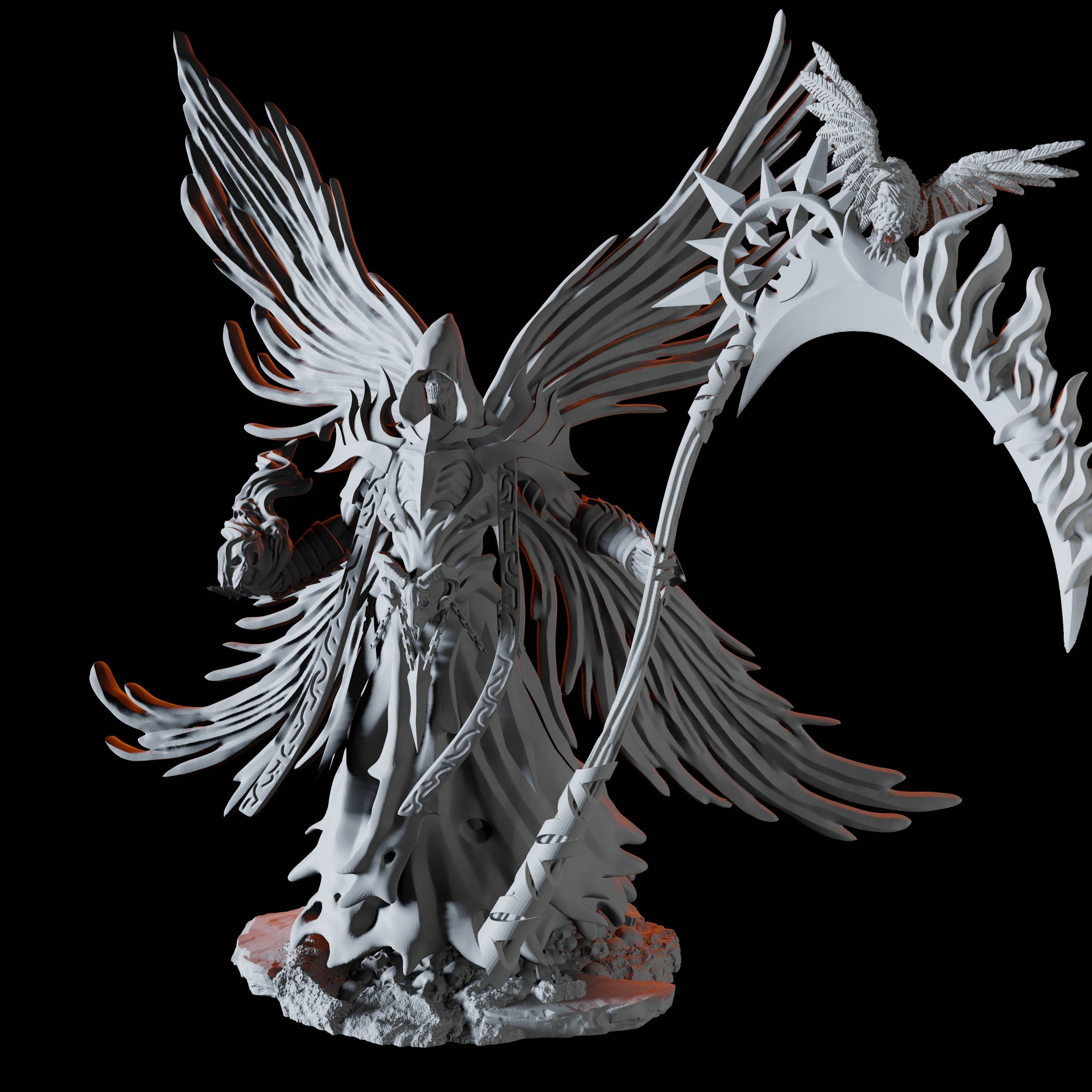The detailed sculpture depicts a fantastical wizard-like figure, crafted in a grayscale palette leaning more towards white with subtle red accents, likely illuminated by red backlighting. Standing against a completely black background, this character exudes an aura of eerie mystique, highlighted by its skeleton face partially obscured by a hooded cloak. The figure wields a weapon in its left hand, resembling a stylized sickle or scythe with flame motifs. Intriguingly, there's a bird perched on this ornate blade. 

The wizard's right hand appears to be gloved or obscured, adding to its enigmatic appearance. Draped in detailed garments, including a notable sash around its neck, the character's attire is intricately designed and emphasizes its imposing presence. Additionally, the figure possesses unique wings that form an X shape, with parts extending downwards, resembling angel wings but with a distinct, otherworldly twist. The entire sculpture is meticulously detailed and set on a pedestal, making it a striking centerpiece that captivates the viewer's imagination.